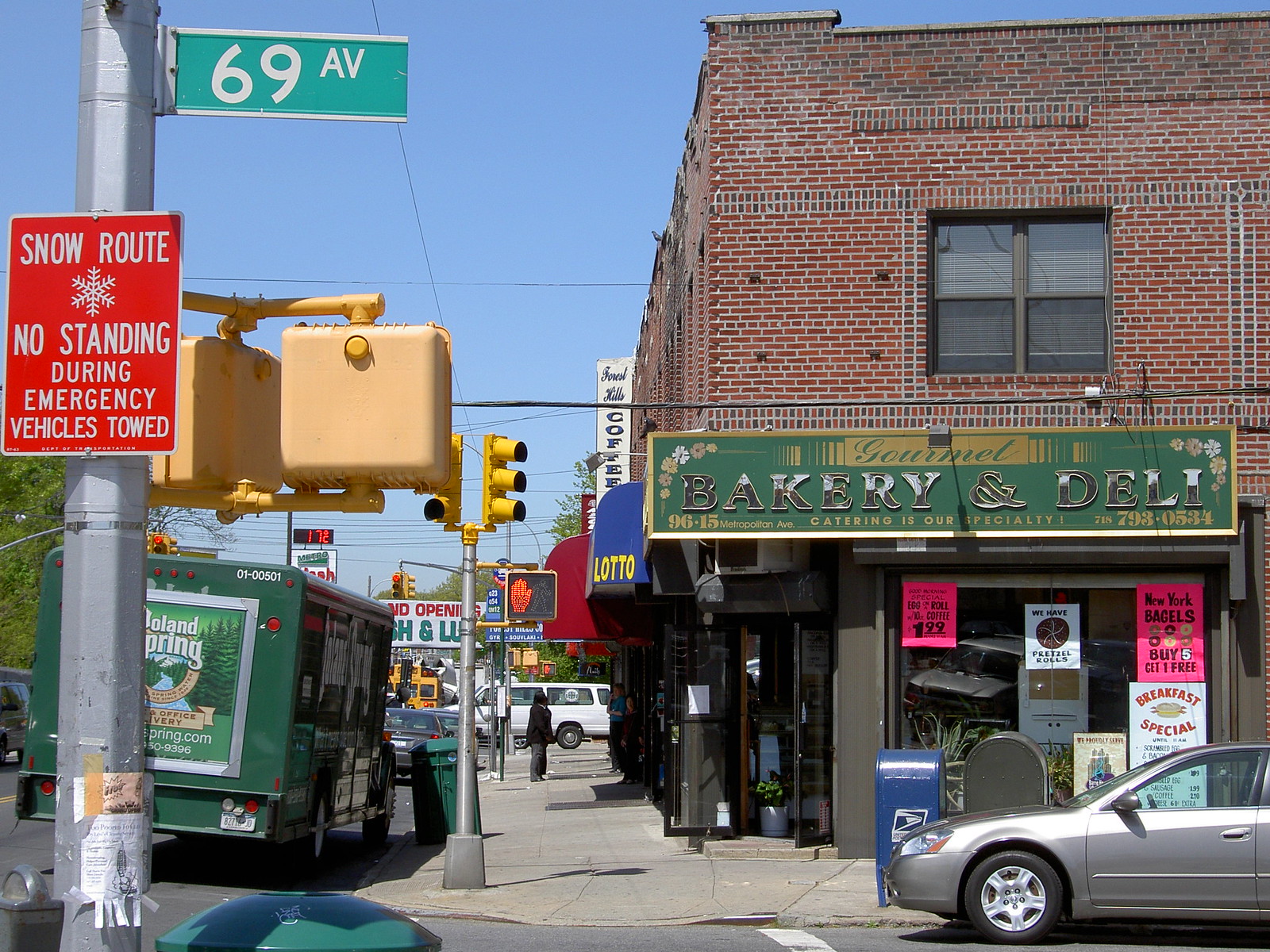This vibrant daytime street scene captures a corner of a small town bustling with activity. Dominating the image is a brick building adorned with a large green sign with silver letters that reads, "Gourmet Bakery. Catering is our specialty." Below, glass doors stand open, inviting patrons into the bakery and deli. The storefront windows are decorated with various signs mentioning bagels and a breakfast special. A red brick sidewalk curves around the corner of the building, where a blue Postal Service mailbox and a gray mailbox stand in front of a gray car parked at the curb. To the left, there's a green Poland Spring truck parked beneath a prominent green street sign that reads "69th Avenue." Above the truck, a red sign warns, "Snow Route No Standing During Emergency Vehicles Towed." Down the street, more traffic, including a yellow school bus, can be seen, while the bright blue sky with no clouds provides a clear backdrop to this lively town snapshot.